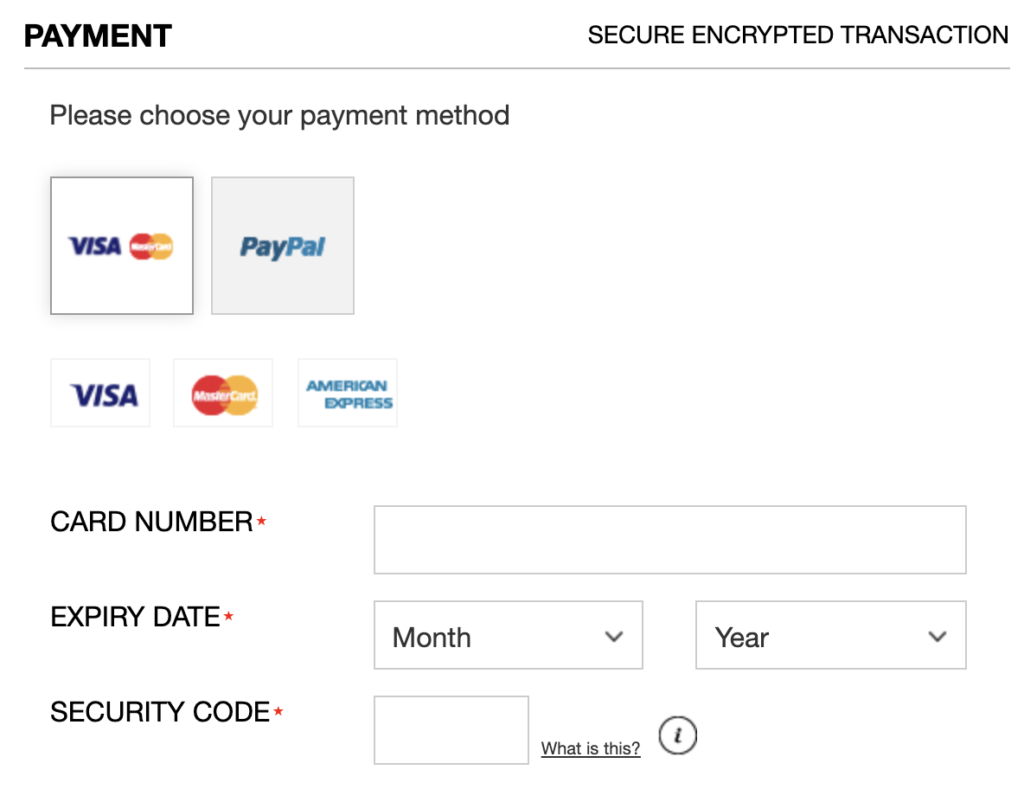The image depicts an online payment page with a minimalistic design featuring a white background. In the upper left-hand corner, the word "PAYMENT" is prominently displayed in uppercase black text. On the upper right-hand corner, the phrase "SECURE ENCRYPTED TRANSACTION" is also in uppercase, emphasizing security.

Below the "PAYMENT" heading, in dark gray text, the instruction "Choose your payment method" is provided. Immediately beneath this instruction, there are several payment logos arranged in a grid: the Visa logo appears first, followed by the PayPal logo, and underneath these, the Visa logo appears again alongside the MasterCard and American Express logos.

Further down, there are user input fields laid out for payment details. The first field is labeled "CARD NUMBER" in uppercase black font, with a red asterisk indicating that this field is required. To the right of this label, there is a box for users to enter their card number.

Below the card number field, there is a section labeled "EXPIRY DATE" (note the uncommon spelling). This section includes dropdown menus to select the month and year of expiration. To the right, there is another required field for the card's security code, accompanied by a small "What is this?" button, which provides guidance on locating the security code.